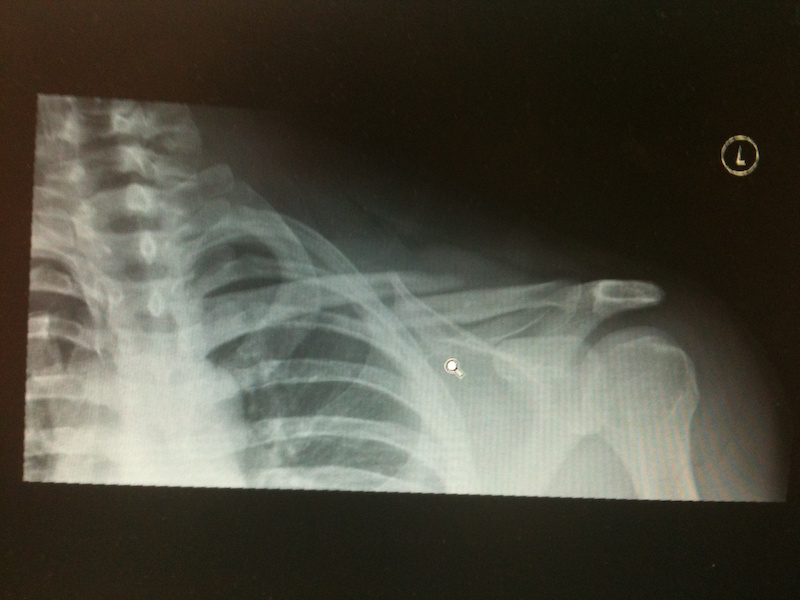The image is an x-ray scan featuring the upper portion of a human torso, focusing on the neck, left shoulder, and partial ribcage. The x-ray, set against a completely black background, is slightly tilted, with the left side positioned higher than the right. The skeletal structures—including the vertebrae, shoulder, and ribs—appear in shades of white to light gray. Notably, there is a cursor image resembling a small magnifying glass located above the bones, indicating that this might be a screenshot taken on a computer. In the upper right corner of the x-ray, a yellow circle with the letter 'L' is visible. This annotated 'L' likely denotes the left side of the torso. Overall, the image provides a detailed view of the left upper thoracic framework, supplemented by digital annotations.